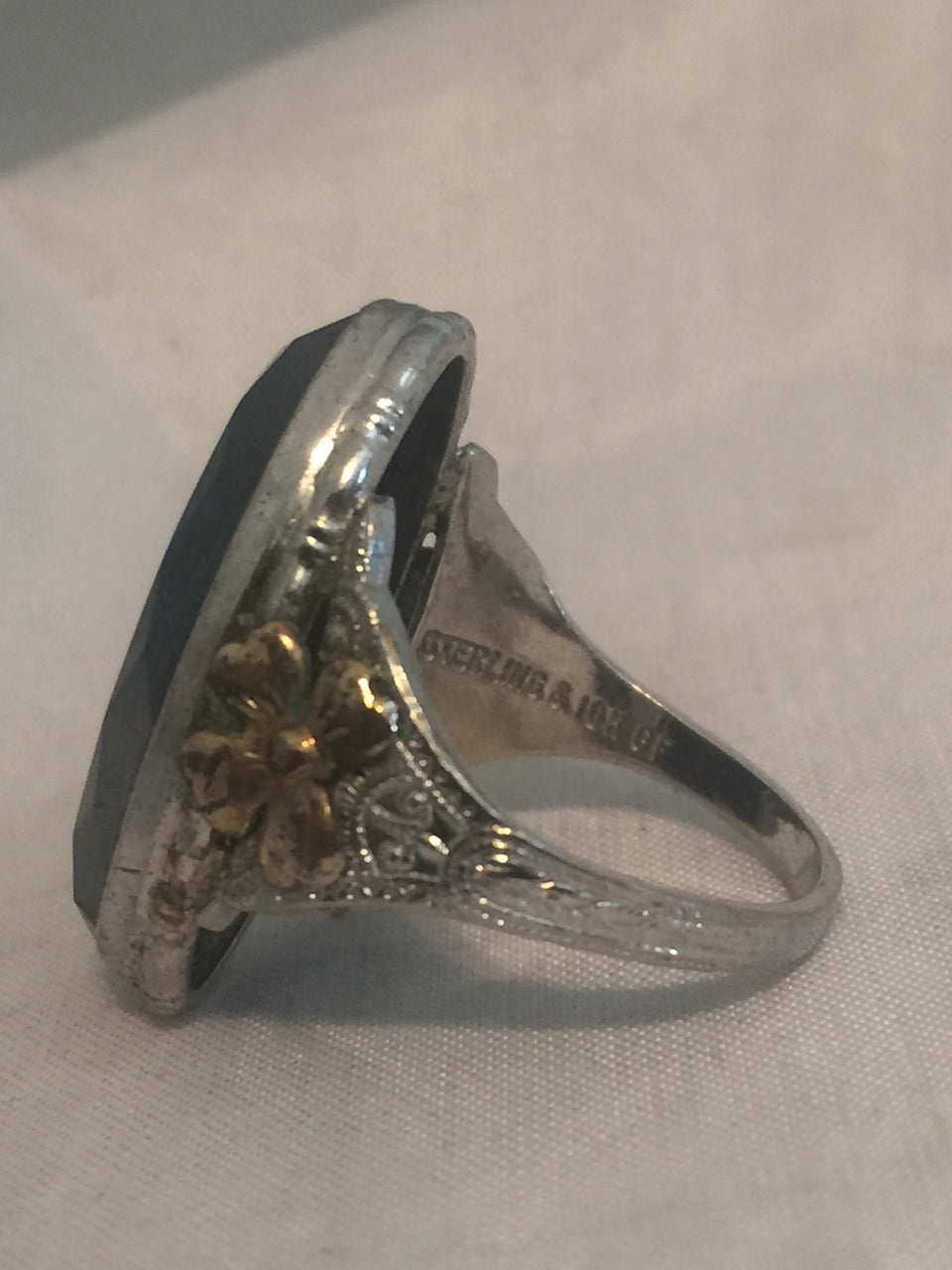The image is a close-up photograph of an old silver ring placed on a white cloth surface. The ring features a narrow band that widens towards the top, showcasing intricate floral and leaf-shaped ornamentation, predominantly gold-colored and slightly darker than the silver. At the center of the ring is a large, dark blue gemstone. The stone appears flat and is centrally set, contrasting with the ornate design of the band. The inside of the band has an inscription, suggesting markings such as "Sterling" and possibly "GF or CF," though the text is not entirely clear. The silver has a slight glow and casts a shadow on the white fabric, adding depth to the image. The photo's overall dark and grainy quality contributes to the perception of the ring being well-worn and aged.